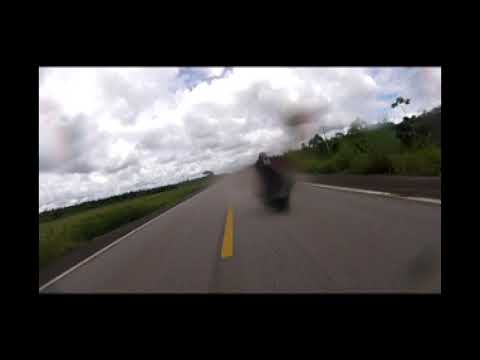An outdoor scene framed in black showcases a two-lane highway cutting through a landscape of fields and trees beneath a cloudy sky. The road, depicted at an upward angle from the mid-left towards the upper right, features white lines on each side and a broken yellow divider line in the center. In the blurry center of the image, a black, indistinct figure, likely a motorcyclist, speeds by, evoking a sense of rapid motion. The muted colors and cloud-laden sky suggest an overcast day, with the sky displaying grey cloud bases and a hint of blue. The left side of the road has tall grass and distant trees, while the right side shows lower vegetation and shrubs. The overall impression captures the fleeting passage of the motorcyclist through this overcast, muted landscape.